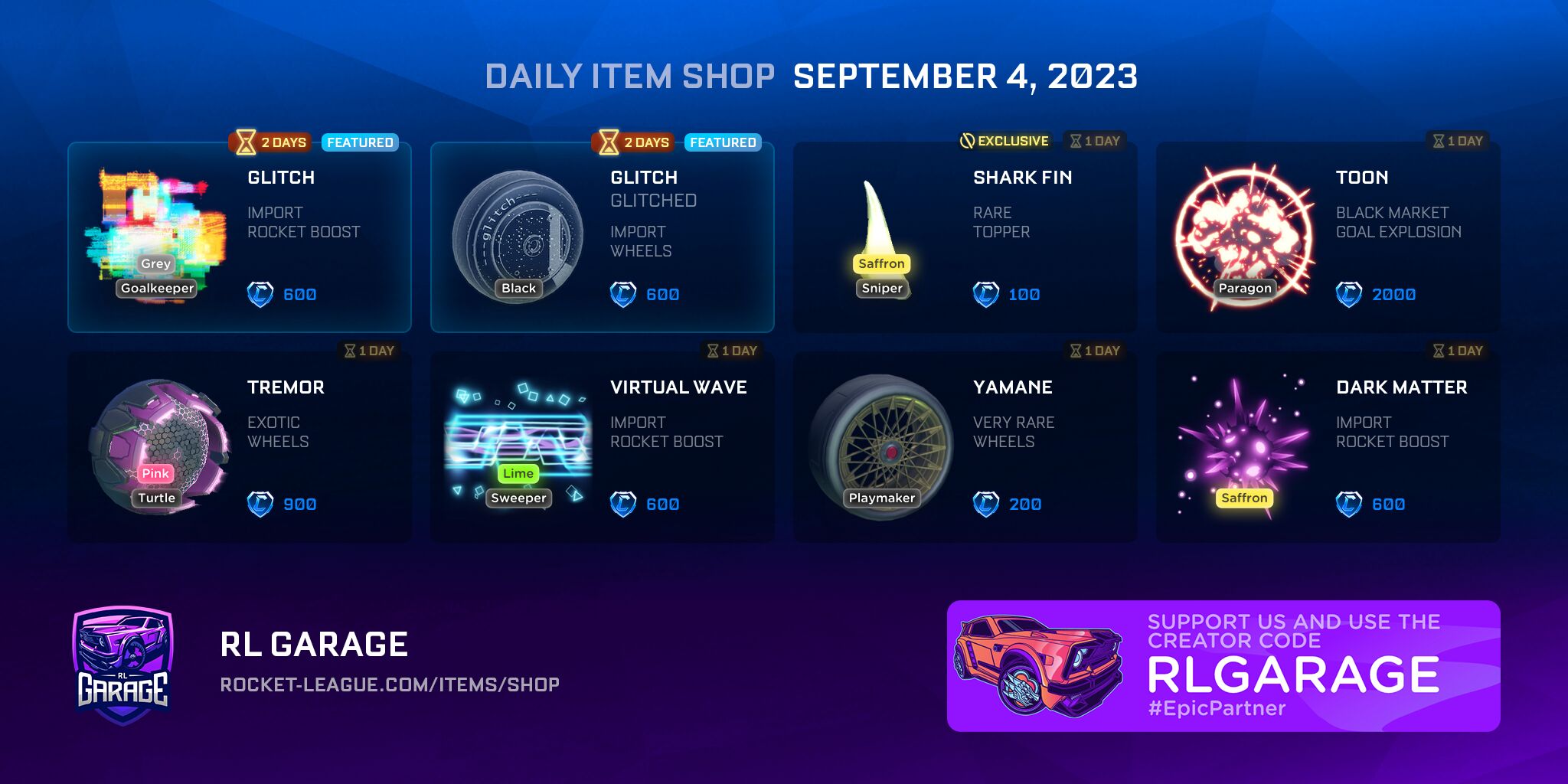This is a screenshot from a video game’s item shop page, labeled "Daily Item Shop" with the date "September 4, 2023" at the top. The shop features a grid layout displaying eight different items for sale, arranged in two rows with four items per row. Each item listing includes the name at the top right, followed by the category, and an image of the item on the left. 

Currently, two items are highlighted: the "Glitch" item, categorized as an Import Rocket Boost, priced at 600 credits (indicated by a "C" icon), and another variant also named "Glitch," which appears to be a type of wheel, also priced at 600 credits. Other items displayed include the "Shark Fin," categorized as a Rare Topper, costing 100 credits, and "Toon," an item priced at 2,000 credits, among others. Each item's price is listed in blue text next to the "C" icon on the right side of the respective entry.